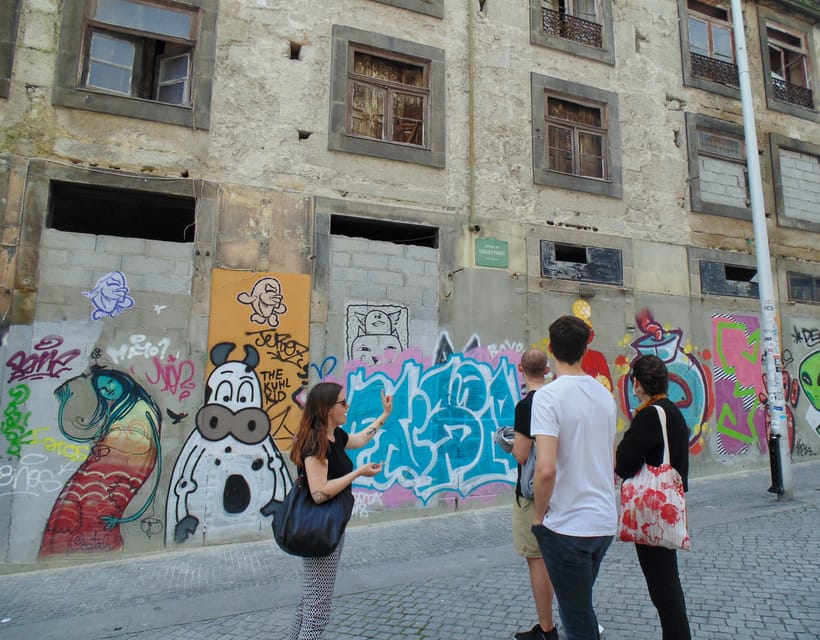In this image, four people are walking on a gray brick walkway towards an old, stone-like building with numerous windows. Three of them, two men and one woman, have their backs to the viewer. The first man wears a white shirt, the woman, sporting a black shirt with a white bag around her arm, and the second man, in the front, has on shorts and a black shirt. A fourth woman, standing to the left, is visible from her right side. She has long black hair, wears sunglasses and a black shirt, and carries a blue bag on her right shoulder. This woman, adorned with tattoos, appears to be pointing and talking to the group as if guiding them or explaining something about the building.

The building in front of them is adorned with vibrant wall art and graffiti, including depictions of a girl, a white cow, text, a grenade, an alien, and what appears to be a mermaid and a vase. Despite its old and distressed appearance, the building still has open windows and terraces, suggesting that it might be inhabited. A large metal pole stands beside the group, marking the cobblestone street on this overcast day with good lighting, creating a scene where the group seems to admire the urban artwork.